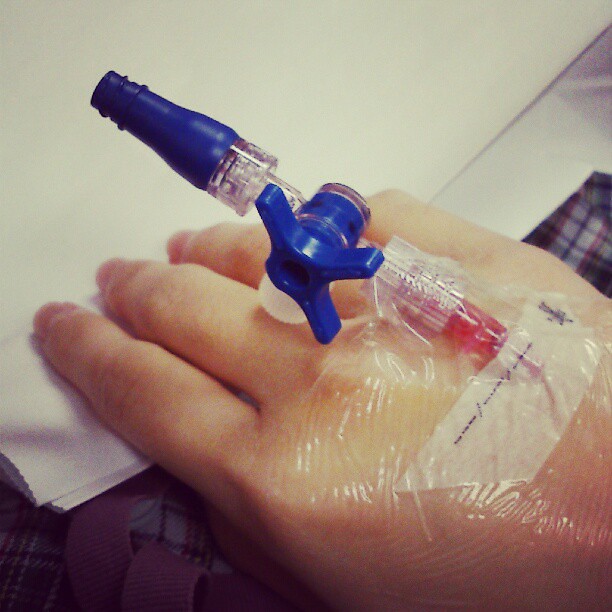The image depicts a detailed medical scene featuring a person's right hand, which is receiving medical attention. The hand is positioned over a pair of flannel pajama bottoms and is grasping white papers with the thumb tucked beneath the four fingers. Clear medical tape secures an IV device on the top of the hand. The IV comprises a blue port and a clear section with a twist knob in the center, allowing fluids to be administered or blood to be drawn. A needle, partially inserted into the hand, reveals traces of watery red liquid, emphasizing the ongoing medical procedure.